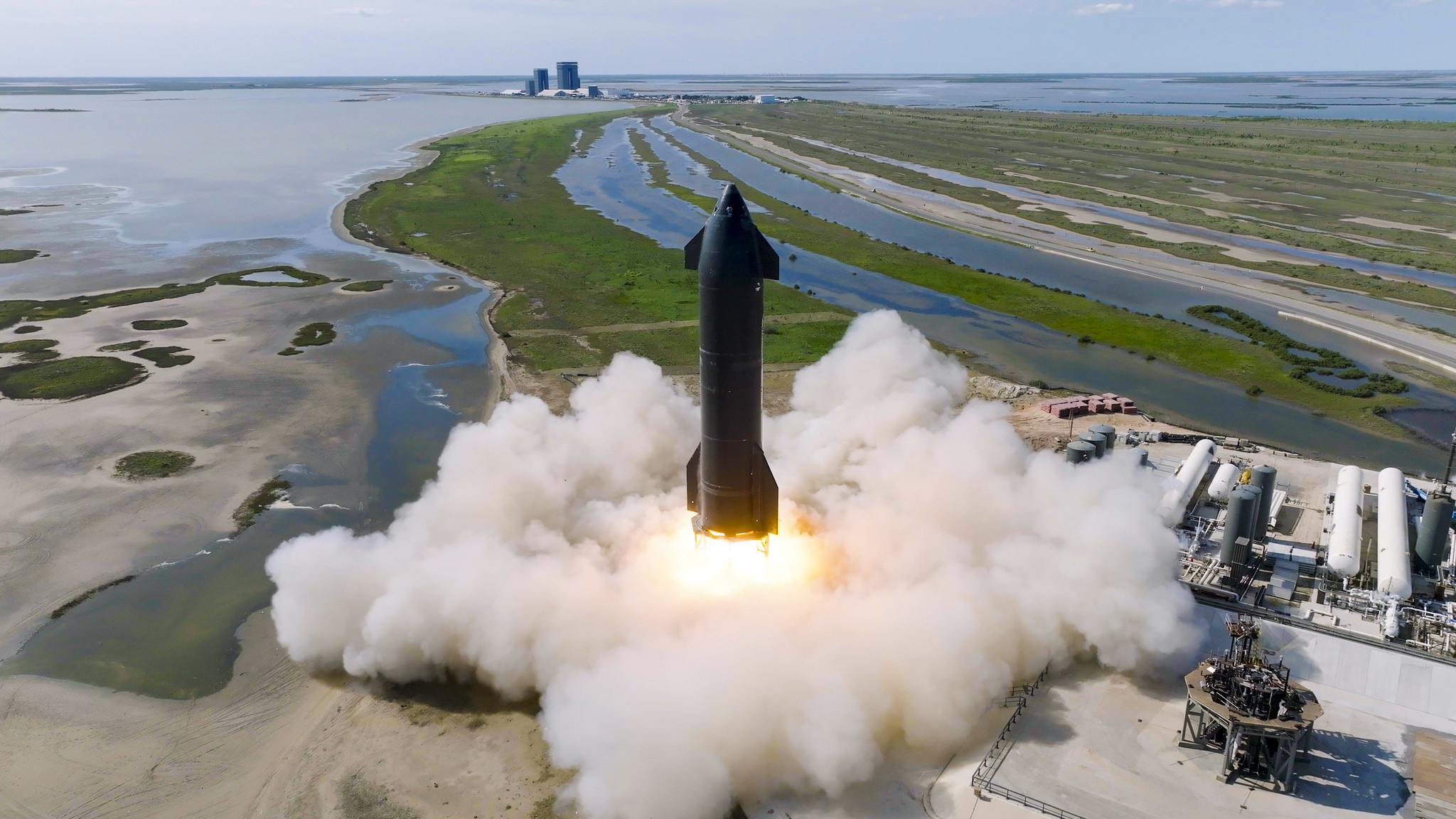This high-altitude drone photograph captures the dramatic launch of a SpaceX Starship rocket, painted in a distinct black color and devoid of any logos. The rocket, prominently positioned at the center of the frame, has just lifted off, generating intense yellow and orange flames at its base. These flames are surrounded by massive plumes of grey smoke billowing outwards. The launch site appears to be a coastal region with extensive wetlands, resembling areas characteristic of Kennedy Space Center or Cape Canaveral in Florida. This similarity is supported by the presence of several tall buildings near the horizon, possibly serving as command centers. Also visible are large fuel tanks in the bottom right corner of the image, including four white ones and a couple of grey. The expansive background consists of a mix of water and wasteland, capturing the stark and isolated beauty of the launch environment.